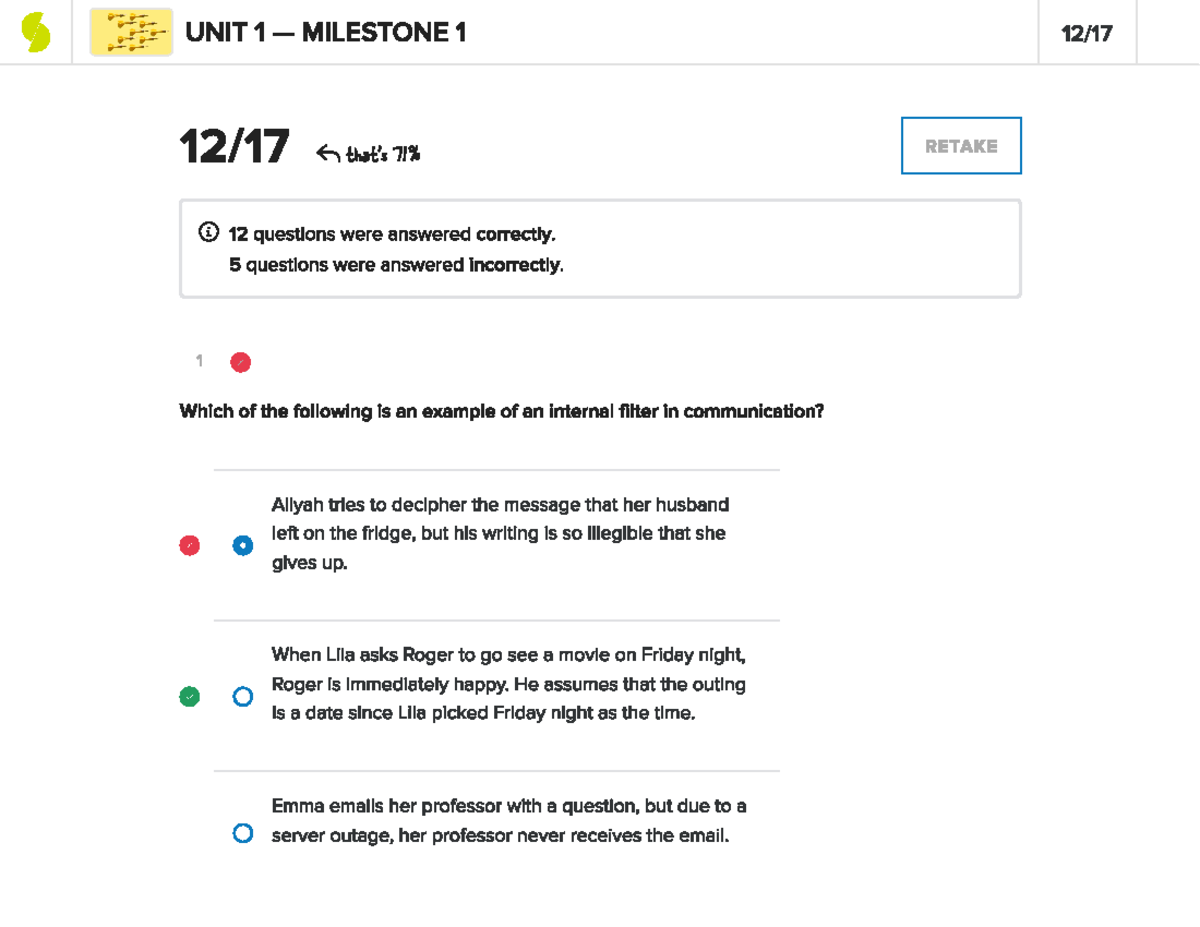The image displays a user interface from an educational app, specifically highlighting "Unit 1 - Milestone 1" in bold text. At the top left, there is a green logo next to a yellow square with markings on it. Below this header, there is an underline separating it from the rest of the content. To the far right, the date "12/17" is indicated, with an arrow pointing to the date and a note that says "bet 7%." Further down, it reads "Retake," signifying an option to retake the test.

The performance details are shown: "12 questions were answered correctly" and "5 questions were answered incorrectly." An example question displayed is: "Which of the following is an example of an internal filter on communication?" Several answer choices are listed below this question, with the incorrect answer highlighted in green, indicating the user's selection.

This detailed interface suggests that the app is designed for educational purposes, allowing users to track their progress and understanding of specific units and milestones through quizzes or tests.